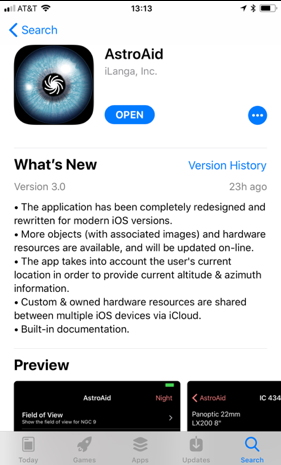The image is a colorful screenshot of a mobile phone displaying an application update screen. At the top, there is a white background with a horizontal black bar featuring the AT&T logo on the left, signal and Wi-Fi strength indicators, what appears to be the time "1330" in the center, and various icons including a battery icon on the right.

Below this bar, in the upper left-hand corner, there is a blue "Search" button accompanied by a back arrow. The app title "Astro 8" appears prominently, alongside a square icon with rounded edges featuring a blue circle and a darker circle with a white galaxy in it, indicating the application's logo. The app developer is listed as "Langia Inc."

Underneath the logo, there is a blue button labeled "Open," followed by three dots in a horizontal arrangement. The text "What's New" is visible beneath this, followed by "Version History" which indicates the current version is 3.0, released 23 hours ago.

The update notes reveal major changes: the application has been completely redesigned and rewritten for modern iOS versions, multiple new objects with associated images and hardware resources have been added, location-based features now provide current altitude and azimuth information, and custom hardware resources can be shared across iOS devices via iCloud. The app also now includes built-in documentation.

A preview section follows, showing two partially visible black screens with white text. The bottom of the image features a grey navigation bar with various phone icons, with the "Search" icon highlighted in blue.